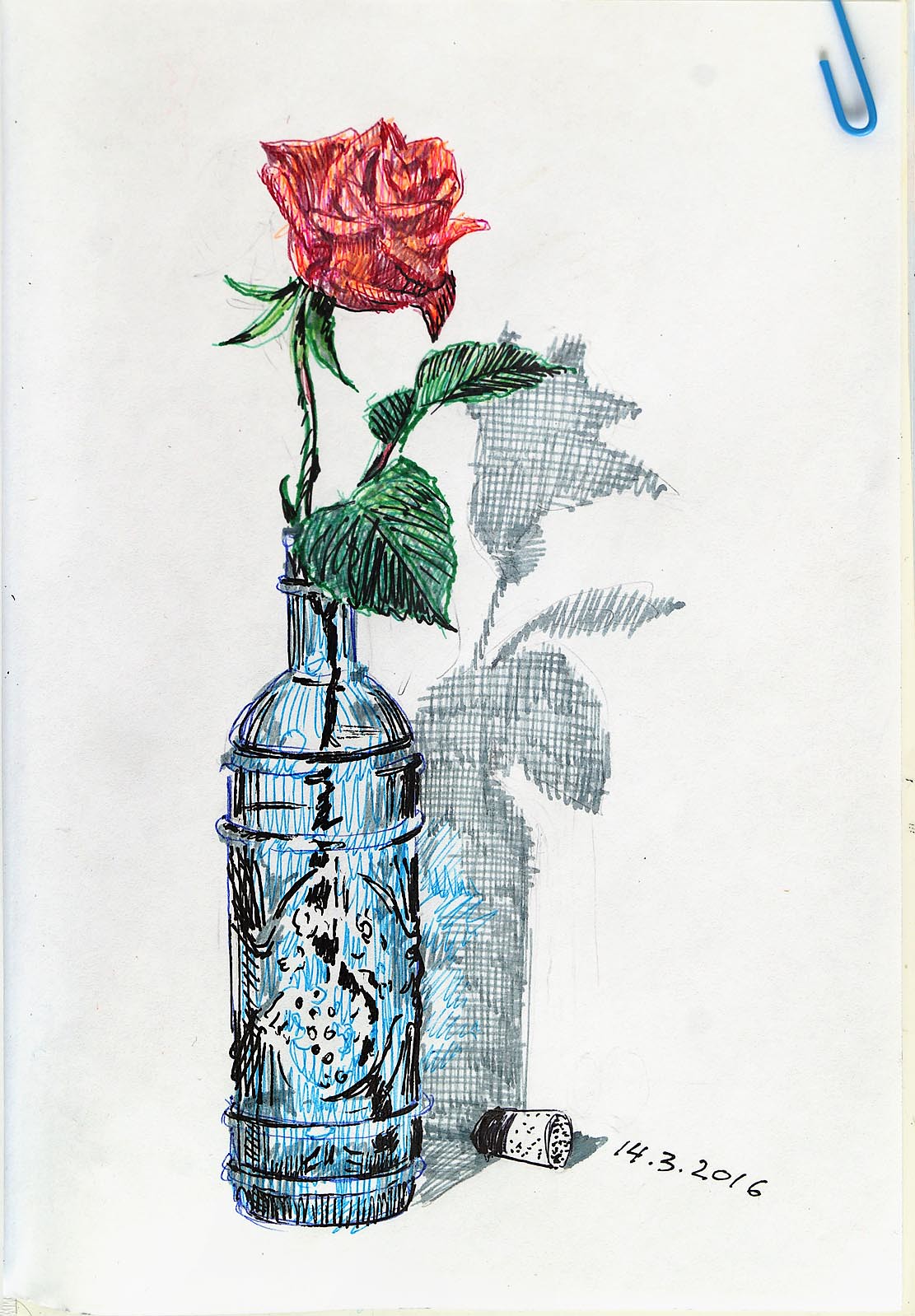This vertical drawing, executed in black pen and ink, exudes intricate detail and thoughtful composition. In the upper right-hand corner, a medium blue paper clip is attached to the paper, adding a touch of spontaneity. The central subject is a clear bottle with a narrow neckline, its surface adorned with subtle black and blue lines that hint at depth and form. Emerging from the bottle is a single rose on a stem, partially opened to reveal its inner structure. The receptacle beneath the bloom is distinctly visible, along with several green leaves.

A second stem protrudes alongside, bearing two green leaves and a central rosebud that remains mostly closed. This bud displays a few layers of petals beginning to unfold. The artist has enriched the composition with a fascinating shadow across the background, employing a pattern of tiny gray squares that lend texture to both the flower and the bottle.

Positioned on the surface below is a sideways cork, engraved with the date "14.3.2016," grounding the artwork in a specific moment in time. This meticulous attention to detail and the interplay of elements create a visually arresting and thought-provoking piece.